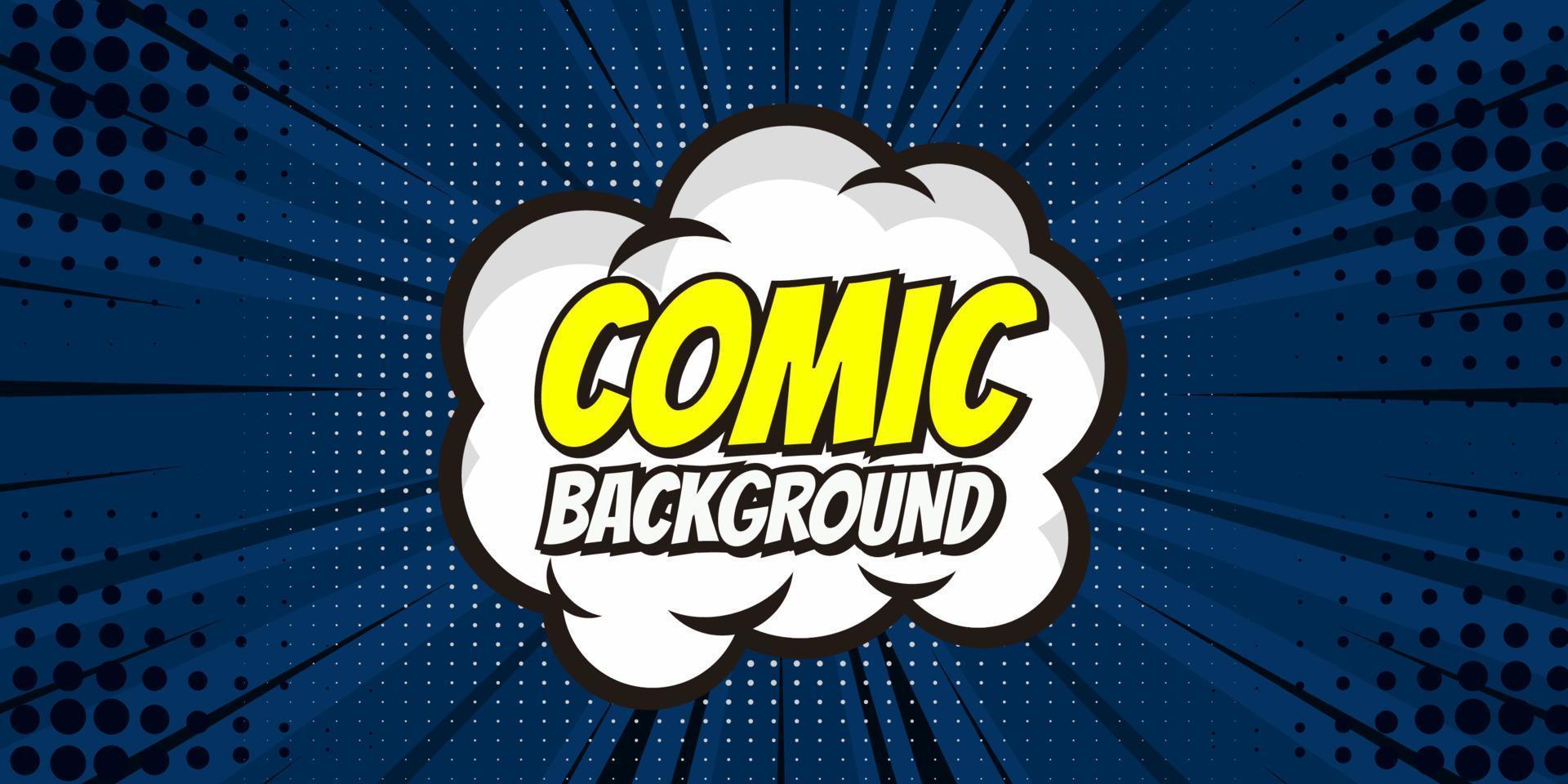This image appears to be an advertisement for a company called Comic Background, featuring a central white cloud with the bolded text "Comic Background" overlaid on it—"Comic" in yellow and "Background" in white, both outlined in black. The cloud, reminiscent of a classic comic book explosion cloud, dominates the center of the image. Surrounding the central cloud is a dark blue and navy striped background, interspersed with various black and white dots and stripes, creating a dynamic and slightly optical illusion-like effect. The overall aesthetic is very cartoonish and flat, typical of comic book art, with the patterns adding visual interest and depth to the otherwise 2D scene.